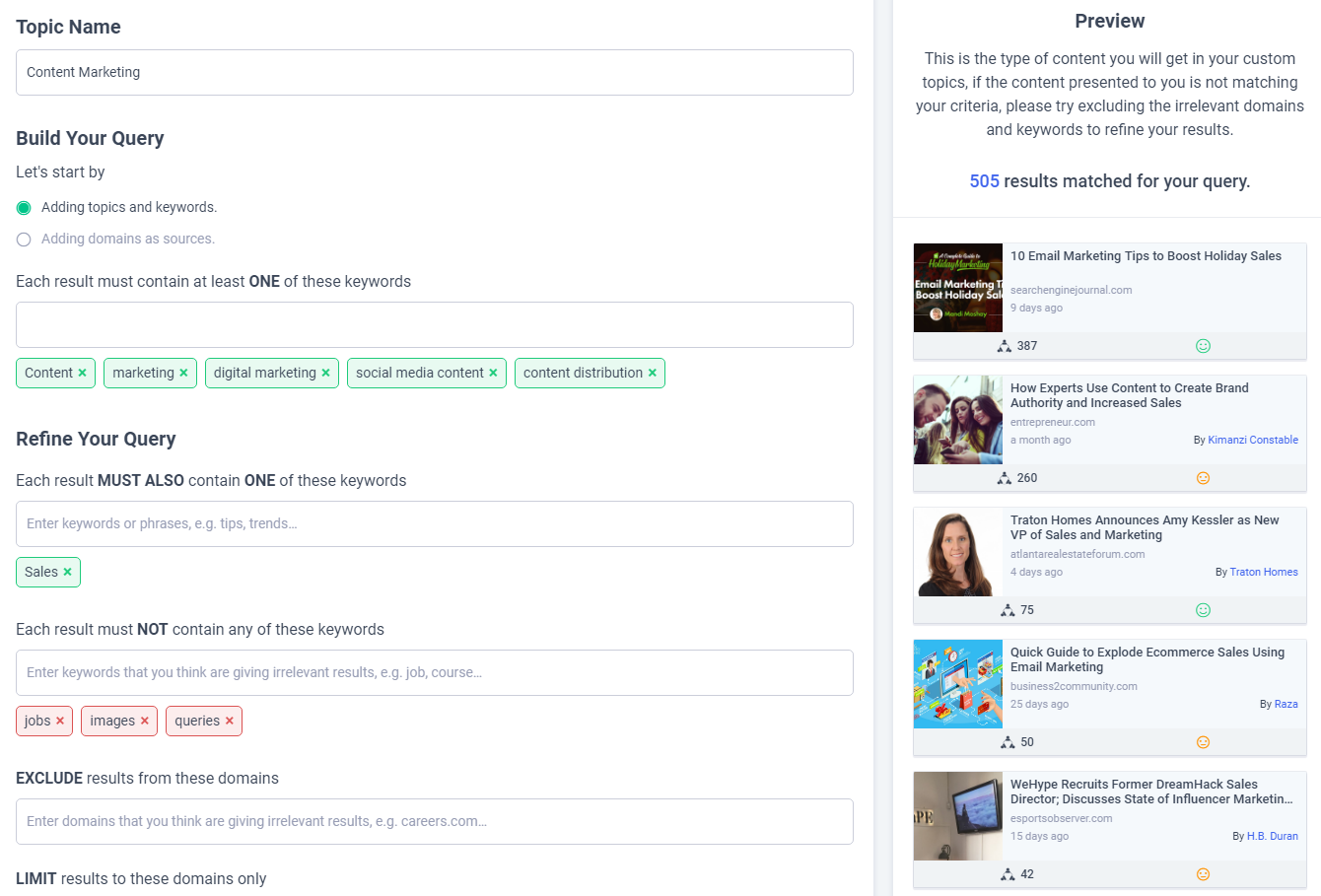This detailed caption describes a website interface designed for creating and refining queries related to content marketing.

---

This image showcases a comprehensive query development interface on a content marketing-focused website. The left-hand side of the page features a series of query-building tools against a clean, white background. From top to bottom:

1. **Topic Name**: A header with an adjacent text box pre-filled with "content marketing."
2. **Build Your Query**: A header followed by two radio buttons allowing the user to choose between "adding topics and keywords" or "adding domains as sources," with the former selected.
3. **Keywords Inclusion**: A label instructing that each result must contain at least one of the following keywords. A corresponding text box is available for user input, below which are four green keyword tags: "content marketing," "digital marketing," "social media content," and "content distribution."
4. **Refine Your Query**: Another header with a label for additional keyword refinement. Below the label is a text box for further keyword entry and a green rectangle containing the keyword "sales."
5. **Keywords Exclusion**: A header indicating keywords that should not be included in any result, followed by a text box for input and three red keyword tags labeled "jobs," "images," and "queries."
6. **Domain Filters**: Headers and text fields for excluding specific domains from the results and limiting results to particular domains.

On the right-hand side of the page, the following elements are present:

1. **Preview**: A header accompanied by explanatory text indicating the type of content users can expect from their custom topics and tips for refining their query.
2. **Results Overview**: A summary indicating that "505 results matched your query."
3. **Top Results**: Five gray rectangles each containing specific content. These include:
   - "10 email marketing tips to boost holiday sales" with an image on the left.
   - "How experts use content to create brand authority and increase sales."
   - "Trayton Homes announces Amy Kessler as new VP of Sales and Marketing."
   - "Quick guide to explode eCommerce sales using email marketing."
   - "WeHype recruits former DreamHack sales director discusses state of influencer marketing."

This interface provides a tailored approach to producing, filtering, and previewing content marketing results based on specified keywords and domains.